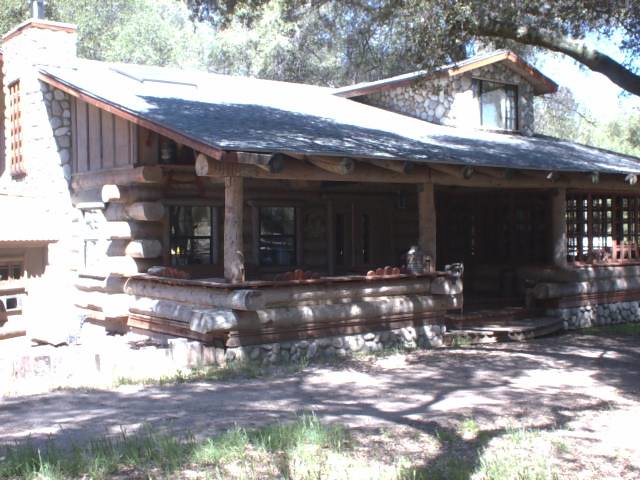This photograph captures a traditional log cabin, constructed primarily from logs, evoking an old-fashioned rustic charm. The cabin appears to be one story with an additional loft, as evidenced by the window embedded in the stone chimney on the roof. The roof itself is wooden, complementing the log exterior of the house. The foundation showcases some intricate stonework, providing a sturdy base. 

A small set of steps leads up to the cabin, suggesting a welcoming entrance. The landscape surrounding the cabin consists of brown dirt with sparse patches of grass, indicating a rugged, perhaps rural setting. The sun casts a warm light over most parts of the house, highlighting its extensive structure which could potentially accommodate up to five bedrooms, hinting at its surprisingly large size.

The photograph is taken from an angle slightly to the left, revealing the chimney on this side. The stone chimney, with visible concrete binding the stones, extends upwards, adding to the rustic aesthetics. Additionally, a prominent tree stretches over the cabin from the right, almost as if sheltering it. This tree not only adds to the picturesque quality of the setting but also reinforces the notion of the cabin being nestled in nature.